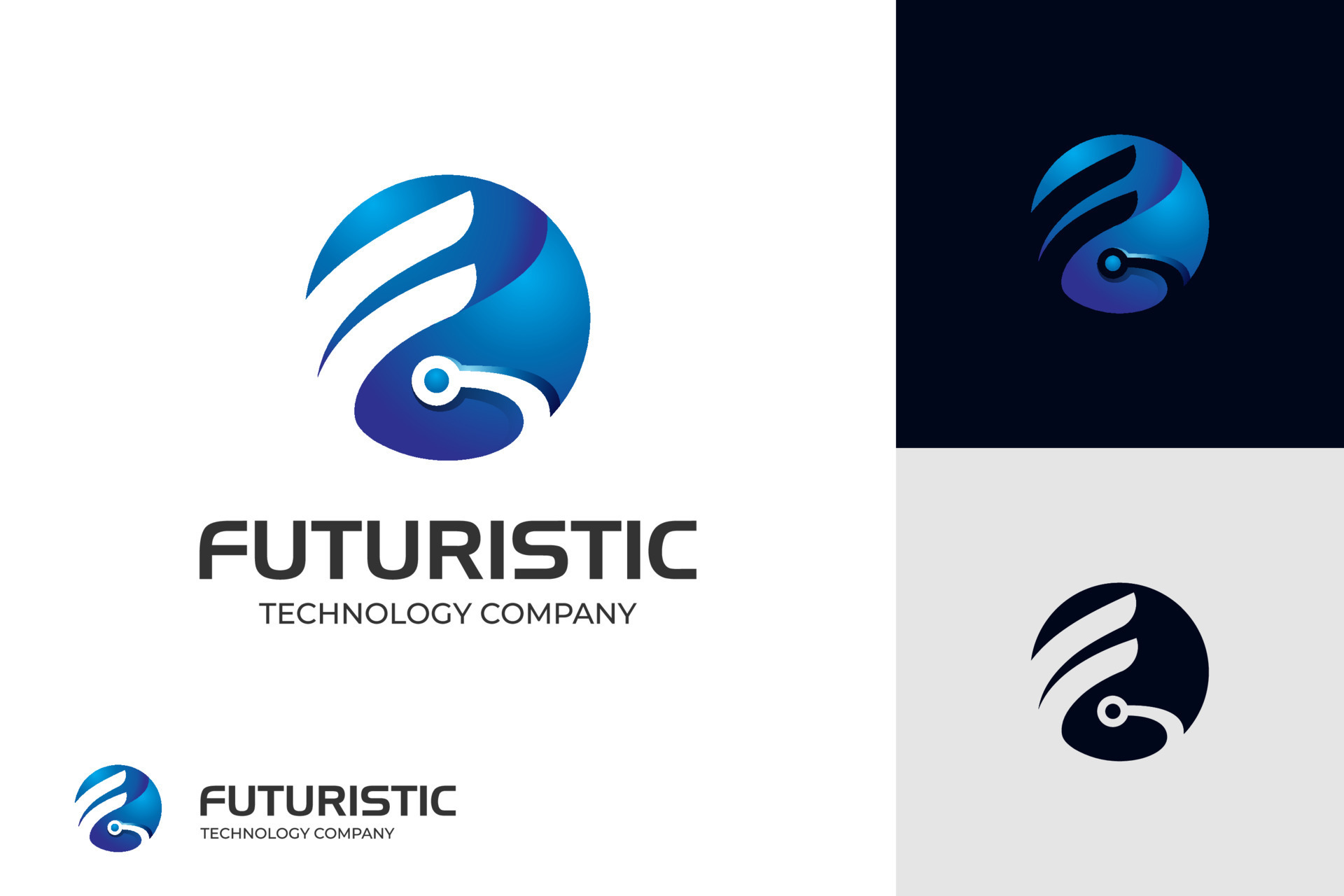The image is a composite divided into three main segments, prominently showcasing the logo and branding of the "Futuristic Technology Company." The central and largest part, occupying over 60% of the image, features a white background with a blue circular logo placed in the upper middle. This logo consists of a blue circle with two horizontal, rectangular oval-shaped protrusions in white, reminiscent of wings or flags, giving it a dynamic and futuristic appearance. Below this central logo, the company name "Futuristic Technology Company" is displayed in bold font.

To the right, the layout is split into two smaller sections. The top right section contains a black background with the same blue circular logo, but the protrusions are black, blending seamlessly with the dark backdrop. Directly below, the bottom right section features a silver-gray background with a navy blue logo, reversing the color scheme and providing a monochromatic variation.

Together, these elements create a cohesive visual representation of the company's brand, highlighting the versatility and futuristic essence of its logo in various color schemes and background settings. Each section reinforces the central theme of innovative technology through consistent design elements and branding.